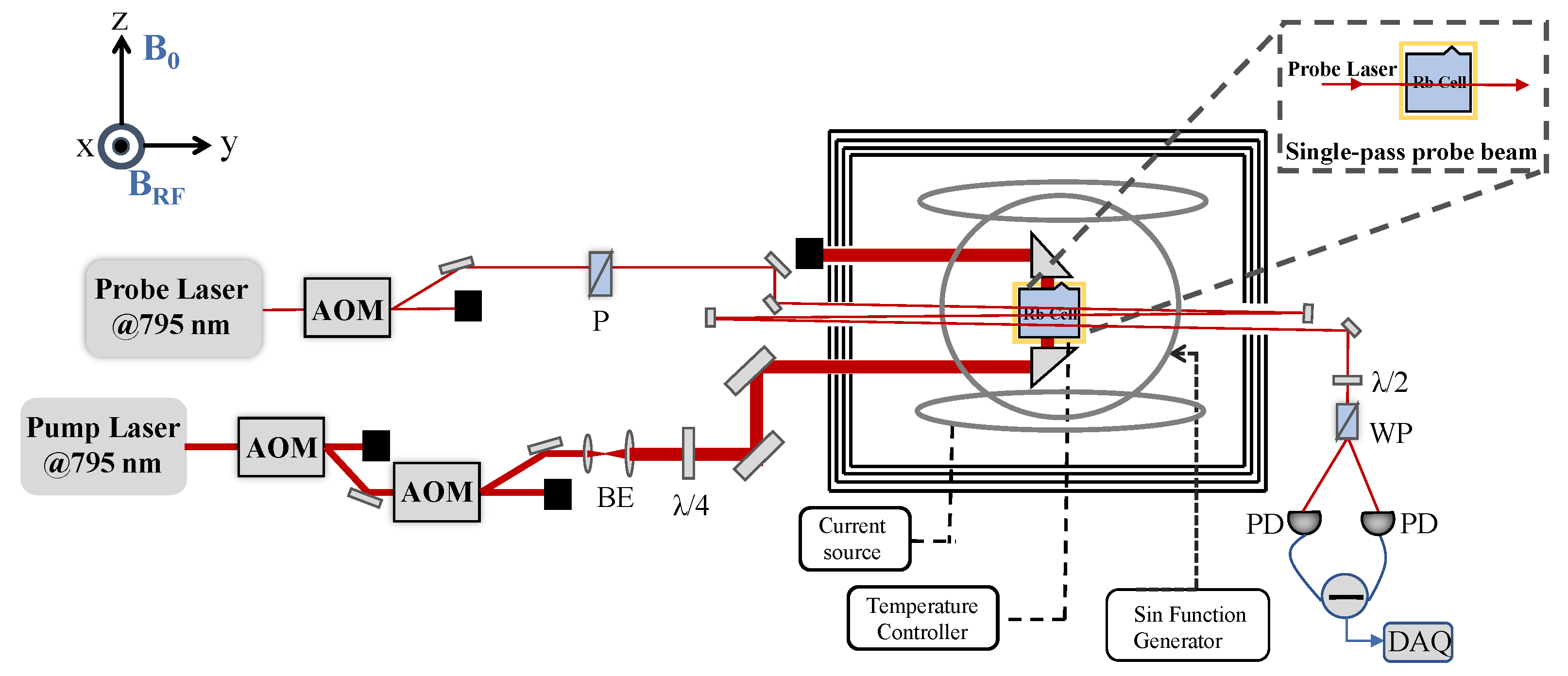The image is a detailed schematic diagram, depicting a laser setup. It starts on the left with two probe lasers, both operating at 795 nanometers, and each leading to a box labeled "AOM" (Acousto-Optic Modulator). These lasers are represented by thin red lines that become thicker as they progress rightwards. 

The setup consolidates in a rectangular chamber featuring two triangular components, highlighted by call-out dotted lines, and centered on a single probe laser beam. Additional elements in this area include a current source, a temperature controller, and a sine function generator. 

Connected to this chamber via red lines are several labels and three small circles arranged horizontally and vertically around a central circle within a square, which has three frames surrounding it. From this central circle, three distinct lines branch out, corresponding to the current source, temperature controller, and sine function generator.

Further annotations include arrows indicating directions with labels 'Z' and 'Y,' and an "L"-shaped arrow connecting them to a point labeled 'X'. Additional labels near various components read "probe laser RB cell single pass probe beam" and "B-R-F". The diagram seems meticulously detailed, emphasizing the connections and interactions between the lasers and other components within the structured setup.